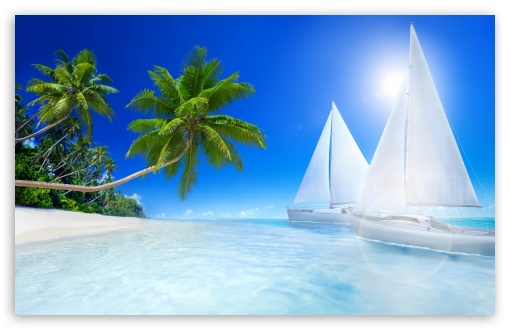The image is a digital artwork in a landscape orientation, depicting a serene tropical coastal scene. The bottom half of the rectangular image, approximately four inches wide by two inches high, features an inviting white sandy beach on the left and crystal-clear, pale aqua-blue water transitioning to a slightly darker hue on the right. Several green palm trees, with their trunks growing horizontally before rising up, stretch over the left portion of the beach, adding a lush, tropical feel. On the right side, two pristine white sailboats with no discernible features or occupants are anchored near the shore, their profiles facing the beach. The sail of the boat on the right almost aligns with a bright, white sun in the clear, brilliant blue sky above, which is devoid of clouds. The overall texture and smoothness of the image suggest that it is an AI-generated graphic design, emphasizing its idyllic and almost surreal quality.